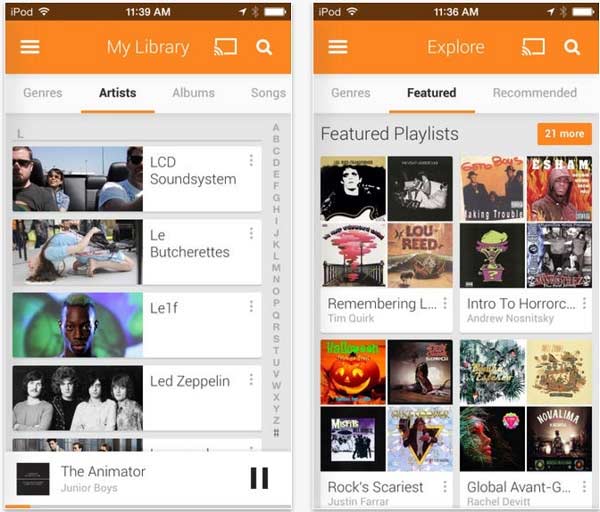The image showcases two screenshots from an iPod library interface. The left screenshot displays the user's music library, while the right captures the 'Explore' section.

**Left Screenshot (My Library):**
- **Header:** "My Library," with an option to cast to a Chromecast.
- **Search Box:** Located beneath the header.
- **Tabs:** Four tabs – Genre, Artist, Albums, and Songs. 
- **Current Tab:** 'Artist' tab is selected.
- **Artist Listing:** Displaying artists under the letter 'L': 
  - LCD Soundsystem
  - Le Butcherettes
  - Lelf (spelled L-E-L-F)
  - Led Zeppelin
- **Alphabet Navigation:** Right side includes an alphabetical navigation list.
- **Currently Playing Track:** "Beat Animator" by Junior Voice.

**Right Screenshot (Explore):**
- **Tabs:** Three tabs – Genres, Featured, and Recommended.
- **Current Tab:** 'Featured' tab is selected.
- **Section Title:** "Featured Playlists."
- **Button:** An orange button labeled "21 more" on the right side.
- **Playlists Displayed:**
  - "Remembering L...," by Tim Quirk (title is cut off).
  - "Intruder Horror...," by Andrew Krasnitsky (title is cut off).
  - "Rock's Scariest," by Justin Farrar.
  - "Global Avant-Garde," by Rachel Devitt.

The detail in the captions allow for a comprehensive understanding of both screenshots, highlighting the functionality and currently displayed content within each section of the app.